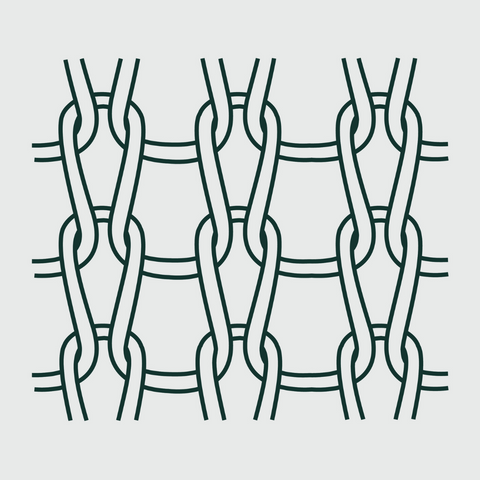The image depicts an intricate black and white chain linkage pattern set against a light gray background. This woven design consists of interlocking loops arranged in a 3x3 grid. Each loop arches at the top and interconnects with the loops on either side and below it, creating a continuous, knotted appearance reminiscent of a complex chain link fence. The stark contrast of the dark loops against the muted backdrop emphasizes the detailed, intertwined structure, which dominates the image without any other elements in focus.